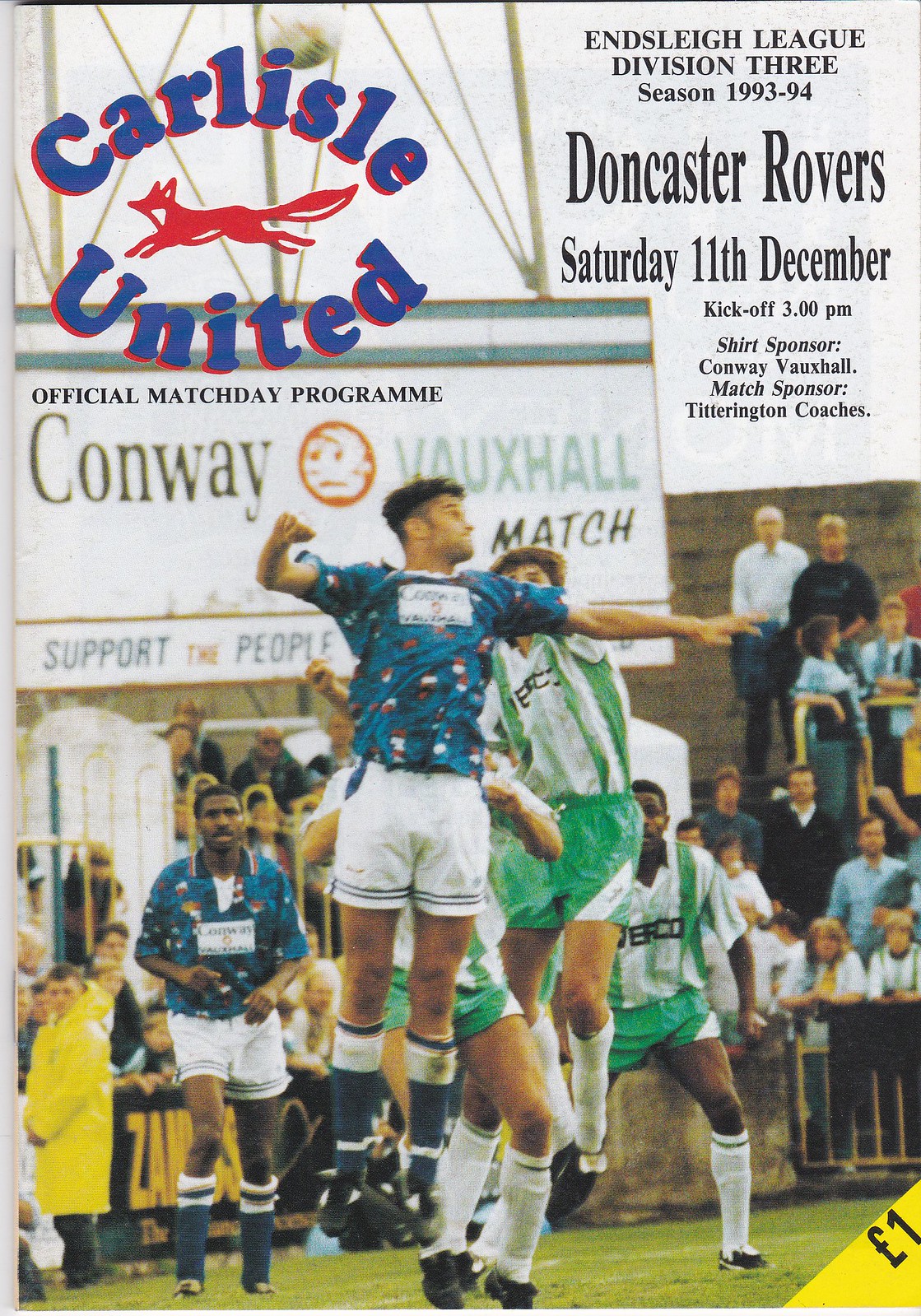The cover of the Carlisle United official match day program for the Enley League Division III season 1993-94 features a vibrant action shot from a football match. Dated Saturday, 11th December, with kickoff at 3 pm, the program previews a game against Doncaster Rovers. The top corners of the cover display "Carlisle United" in blue font with a red outline beside a fox icon. Below this, details of the shirt sponsor Conway Vauxhall and match sponsor Titterington Coaches are listed. 

The central image captures the intensity of a play with a Conway player in a blue, red, and white spotted jersey with white shorts, leaping with a clenched fist, presumably preparing to strike the ball. Behind him, players in green and white jerseys leap alongside, adding to the dynamic energy of the scene. Another Conway player trails just behind. The backdrop features a bustling crowd both standing and seated, adding to the lively atmosphere. In the bottom right corner, the price is marked at £1, embossed in yellow.